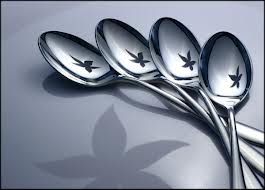This black-and-white stylized image, which appears either AI-generated or painted, features four shiny silver dessert spoons against a monochromatic background. The spoons are arranged with their heads facing forward and tightly clustered at the top of the photograph, overlapping slightly. Each spoon head is adorned with a small, black star-like engraving, resembling a five-pointed leaf or flower petal cluster. The handles of the spoons are intertwined and bent towards the bottom right corner of the image, giving the impression of flower stems.

A faint shadow mirrors this floral design beneath the spoons, extending out of the frame so that only a few petals and leaf points are visible. This detail, along with subtle variations in the monochrome shades—darker corners at the left, bottom, and upper sections of the image—adds depth and complexity. The spoon faces and some portions of their stems seem illuminated, enhancing the reflective quality of the silver and adding a touch of elegance to the composition.